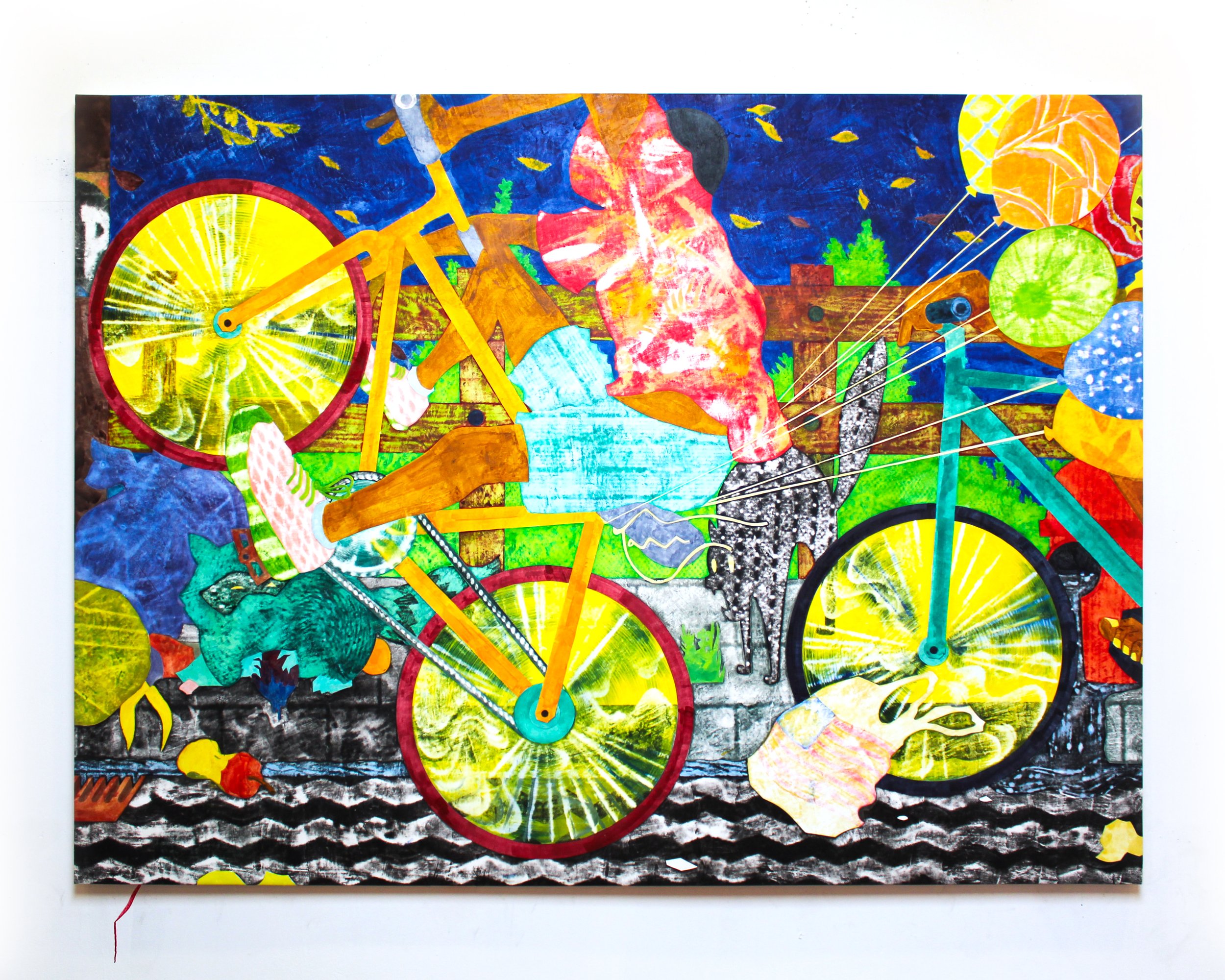The vibrant painting depicts a dynamic scene where a woman, dressed in a Hawaiian shirt with blue shorts and pink shoes featuring a pink grid pattern, performs a wheelie on a brightly colored bicycle with an orange frame, yellow wheels, white spokes, and red tires. Behind her, another bicycle with a turquoise frame and black wheel is partially visible. The surreal setting features a night sky painted in an indigo blue, dotted with green, orange, and yellow balloons, as well as yellow leaves seemingly floating through the air. The ground below them appears abstract with jagged black and white squiggles resembling an angular street. A scared cat with an arched back and raised fur adds a whimsical touch as it stands near the back bicycle. In the background, green trees and grass add a touch of nature to the fantastical scene, while a plastic shopping bag drifts across.